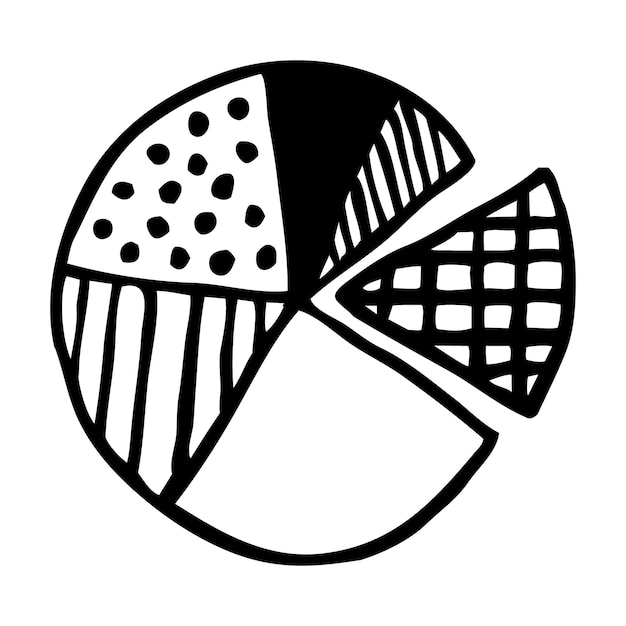The image showcases a striking black and white artwork set against a plain white background with no visible borders. Dominating the center of the composition is a circle measuring approximately three inches in diameter. This circle is meticulously divided into six uneven slices, with one slice noticeably displaced to the right, resembling a piece of pizza. The relocated slice features black horizontal and vertical lines intersecting to form a grid of hollow white squares. Within the remaining circle, the bottom middle slice is completely hollow, presenting a stark, plain whiteness. Adjacent to it on the left, another slice displays vertical stripes slanted slightly to the right. Above this, a segment is adorned with black dots. The two smallest slices, situated opposite each other, include one that is entirely black and the other marked by diagonal lines slanted to the left. This intricate design, with its varied textures and meticulous arrangement, highlights the contrast and complexity within the monochromatic palette.